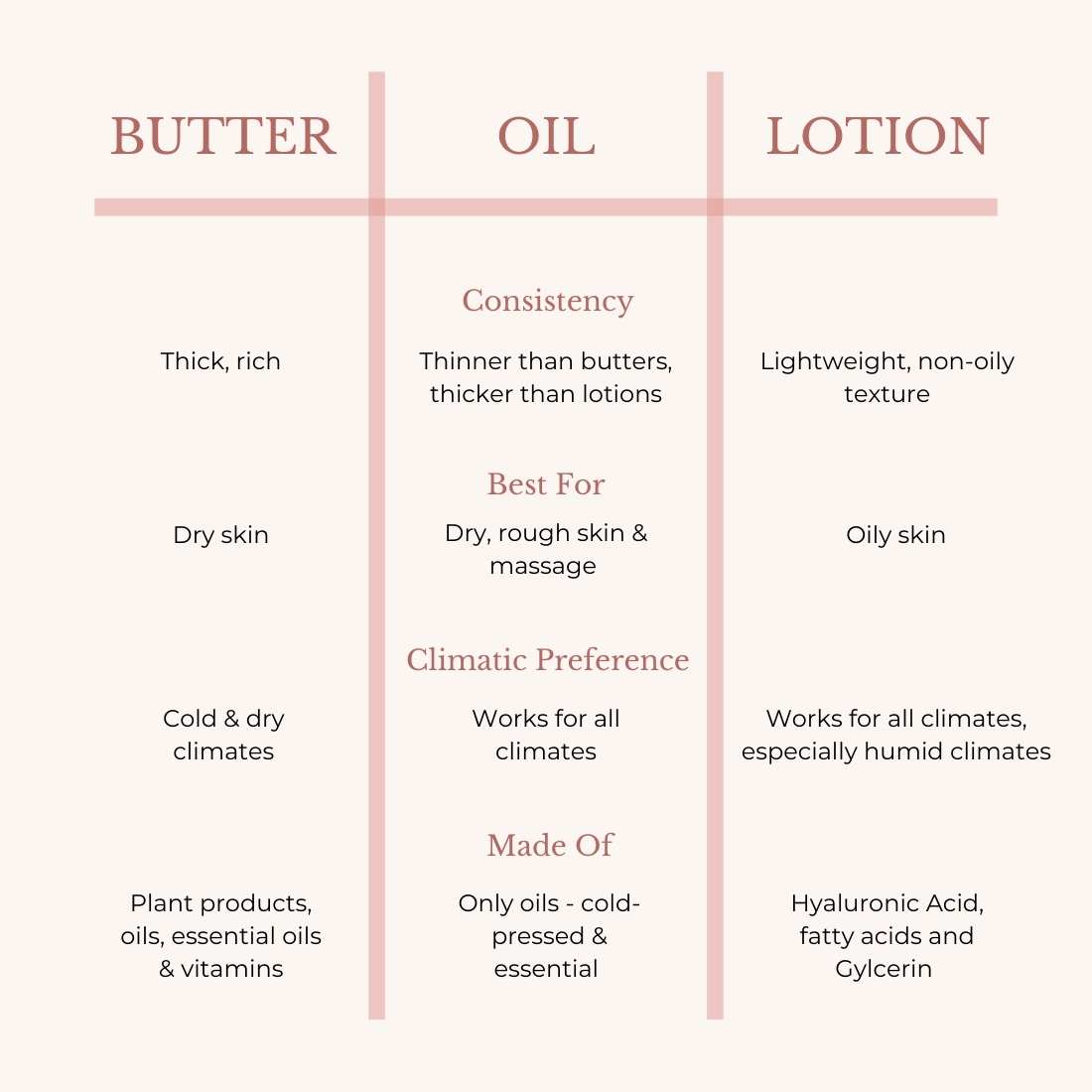This Instagram post features a detailed comparison poster, neatly divided into three columns labeled "BUTTER," "OIL," and "LOTION." Set against a very light pink background with dark pink lines forming a grid, akin to a mini Excel spreadsheet, the headings are in a serif font, all caps, and light brown color. Each column delves into four categories: Consistency, Best For, Climatic Preference, and Made Of.

For "Butter," the poster highlights its thick and rich consistency, making it ideal for dry skin in cold and dry climates, and it is composed of plant products, essential oils, and vitamins. The "Oil" column notes a consistency that is thinner than butter but thicker than lotion, best for dry, rough skin and massages, suitable for all climates, and made from pressed items and essential oils. The "Lotion" column describes it as having a lightweight, non-oily texture, suitable for oily skin.

Overall, the poster succinctly conveys 16 sections of information about these three skincare products, visually organized and easy to reference.